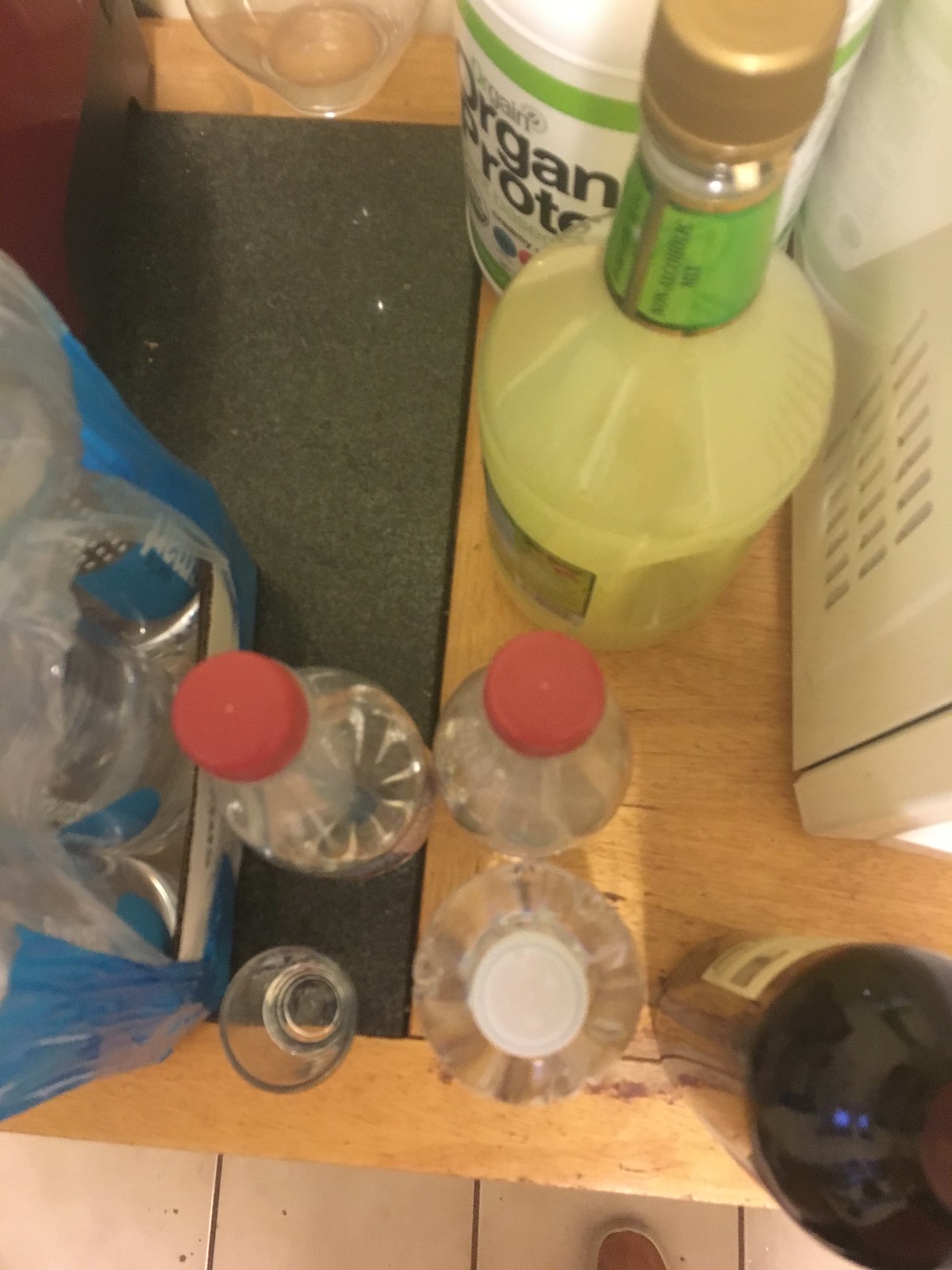This color photograph captures a top-down view of a cluttered kitchen counter made of wooden planks. Centrally placed is a bottle of margarita mix filled with a light green fluid. Adjacent to it is a plastic jar labeled "organic protein" meant for protein shakes. To the side, there's a clear glass drinking cup and an empty shot glass. A blender or similar kitchen device is partially visible. Scattered around the scene are several plastic water bottles, including a pair with red caps and one with a white cap. A large case of mineral water bottles, wrapped in blue clear plastic, takes up the background space. Additionally, a wine bottle appears near the lower corner, opposite the edge of someone's shoe just visible at the bottom of the frame. All these items are tightly packed together on the counter, suggesting preparations for making a drink.